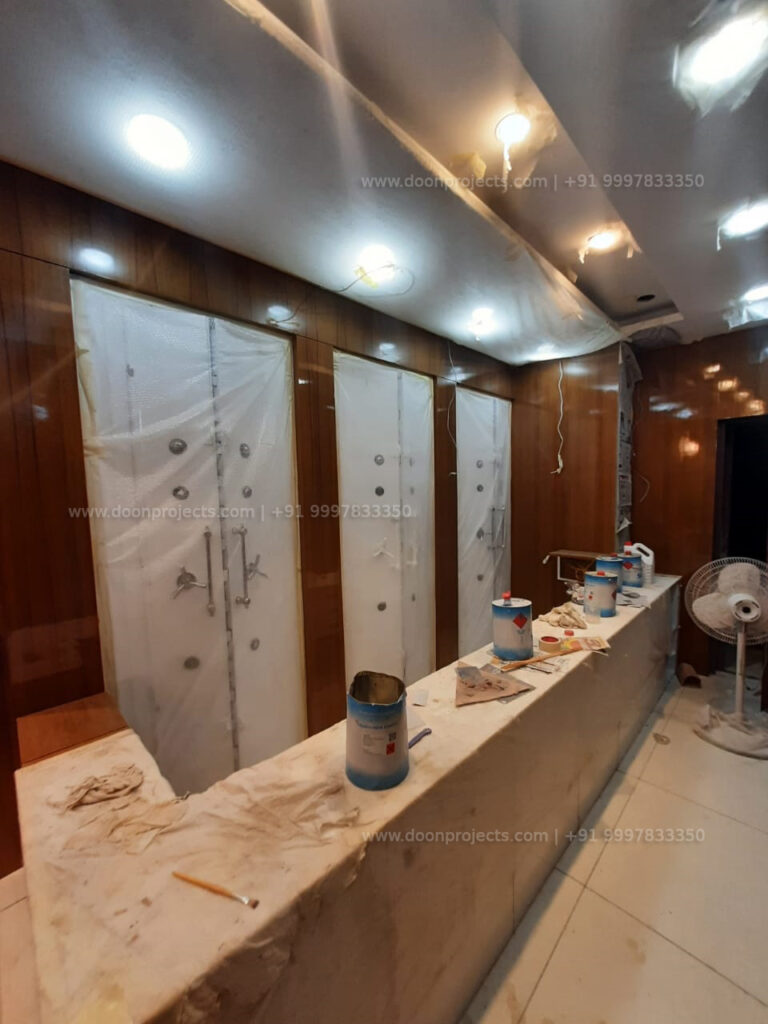The image depicts an indoor construction or renovation scene with key elements being a mix of wood paneling, white tiles, and various construction materials. The ceiling is white, outfitted with recessed lights partially covered by some protective material. A long wooden counter stretches from the bottom left to the center-right of the image, cluttered with blue and white paint cans, pencils, and other miscellaneous items, with some wrapped in white paper. Above the counter, along the left side, is a brown paneled wall featuring three double doors covered in plastic. These doors have long vertical silver handles.

Below the counter, a white tile floor with large tiles is visible, running from the lower right to the center right of the image. Next to the counter on the right side, a white oscillating floor fan is positioned near a black doorway. In the center of the image, the text "www.duneprojects.com" along with some numbers is faintly visible. The scene combines elements suggesting ongoing construction or setup, potentially in a craft store or similar establishment.